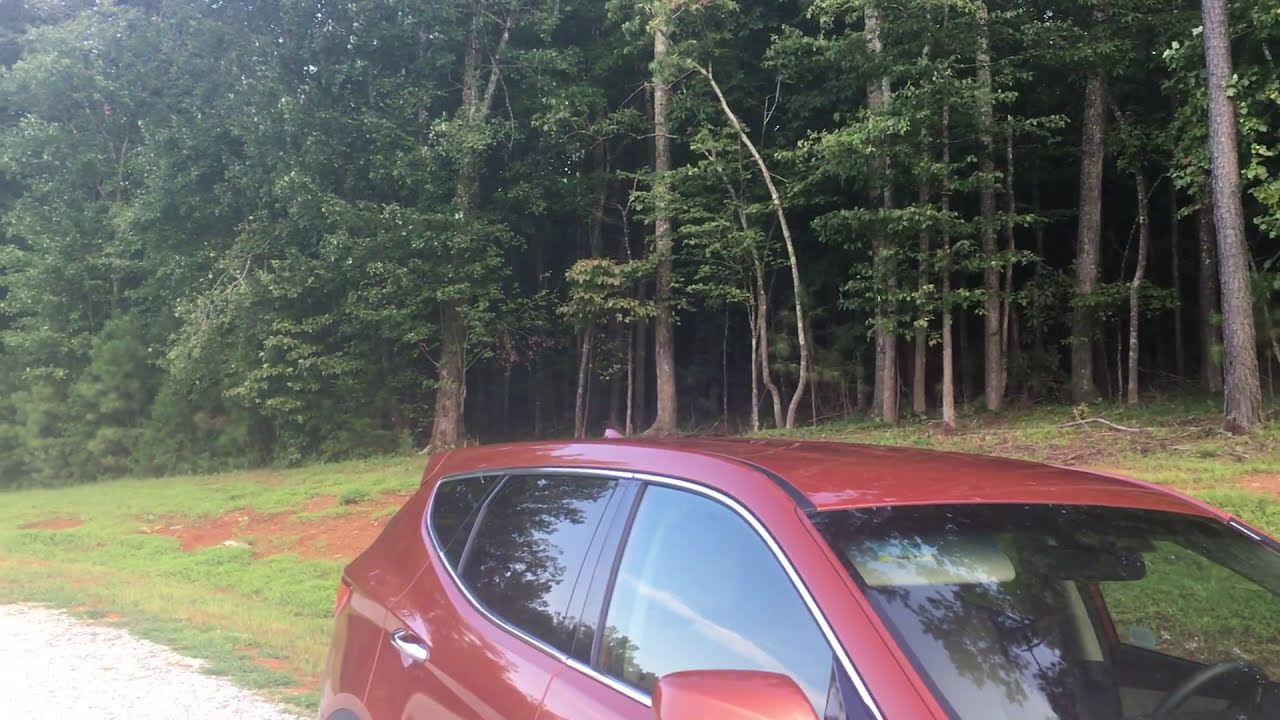The image captures a red Hyundai Santa Fe parked on an unpaved road, situated in the bottom right corner. The car's back side windows are tinted, and the front side window reflects the sky. The setting appears to be outdoors, likely in the middle of the day during spring or summer. The background features a grassy field with patches of red clay-like soil and mud, and behind this field stands a semi-dense forest. The trees on the right are tall and densely packed, with numerous trunks and leaves, while the trees on the left are shorter and slightly less dense, allowing a small portion of the sky to peek through. The overall scene is observed from the perspective of someone standing on the same unpaved road where the car is parked.